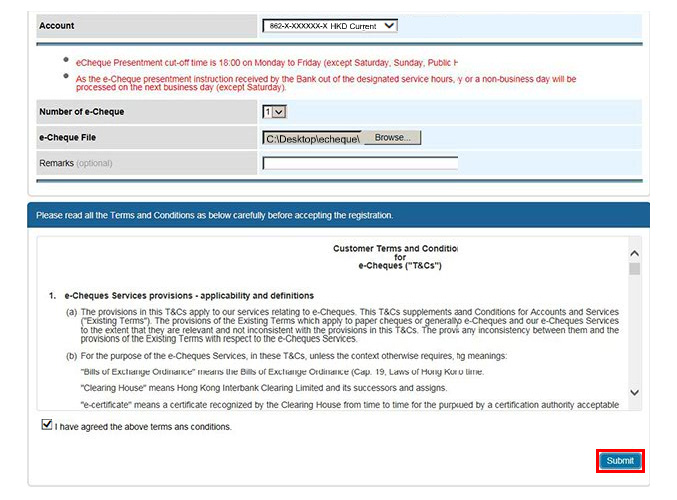This image is a screenshot of a banking application interface. At the top, the word "Account" is displayed in black text on a gray background. Adjacent to this, there's a drop-down menu showing a partially obscured account number, labeled as "892X-XXXXX". Directly below, a section on a white background features red text with two bullet points.

Underneath, there are three gray rectangles labeled "Number of eCheck", "eCheckFile", and "Remarks". The "Number of eCheck" field has a drop-down menu with the number '1' selected. The "eCheckFile" field has a browse button next to it, with a filepath to a desktop location. The "Remarks" field provides an open text input section for user comments.

Further down the interface, a blue rectangle titled "Please Read All Terms" precedes the main section labeled "Customer Terms and Conditions". Here, a list begins with "1. eCheck Services, Provisions, Applicability, and Definitions". Below these terms is a checkbox for users to agree to the terms and conditions.

At the bottom-right corner of the window, a blue "Submit" button is prominently displayed, offering the user an option to finalize their actions.